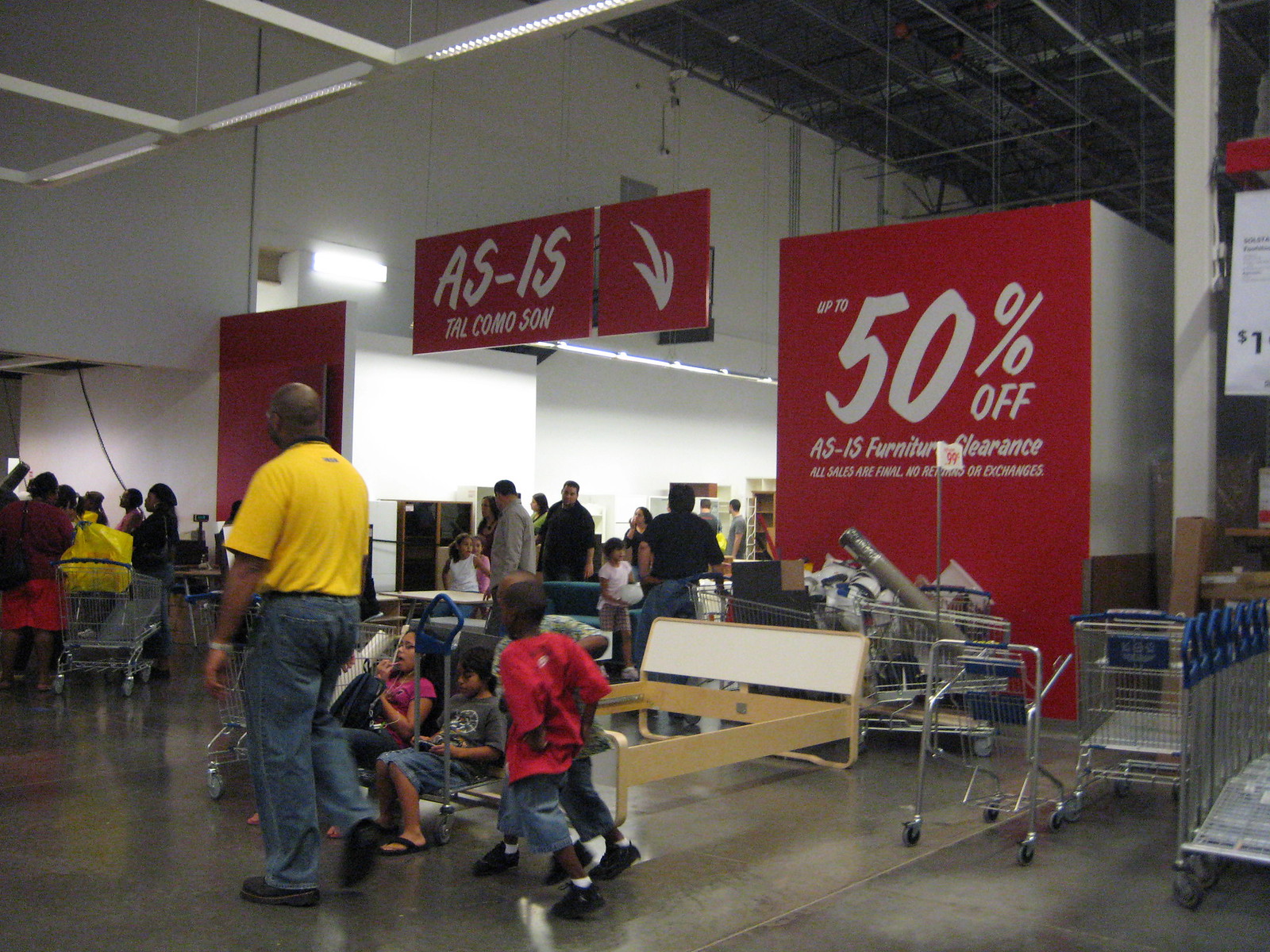This image captures the bustling front area of a large indoor furniture superstore undergoing an as-is furniture clearance event, prominently advertised by a giant red sign in the background indicating "Up to 50% Off" in white letters. The high-ceilinged warehouse features exposed metal beams and is lined with white walls and gray linoleum floors. A sea of shopping carts with blue handles is seen to the right, while numerous shoppers congregate in lines stretching across the middle and left side of the image. Dominating the foreground, a black gentleman dressed in a yellow shirt and jeans, with a watch on his wrist, stands with his back to us, accompanied by a group of children—a boy in red shorts, another in a green shirt, a little boy sitting down, and a girl donning a pink shirt. The scene is teeming with activity as people navigate the crowded space, with some signs denoting all sales are final, no refunds or exchanges, amidst the jumble of tangled shopping carts and the mass of eager shoppers.